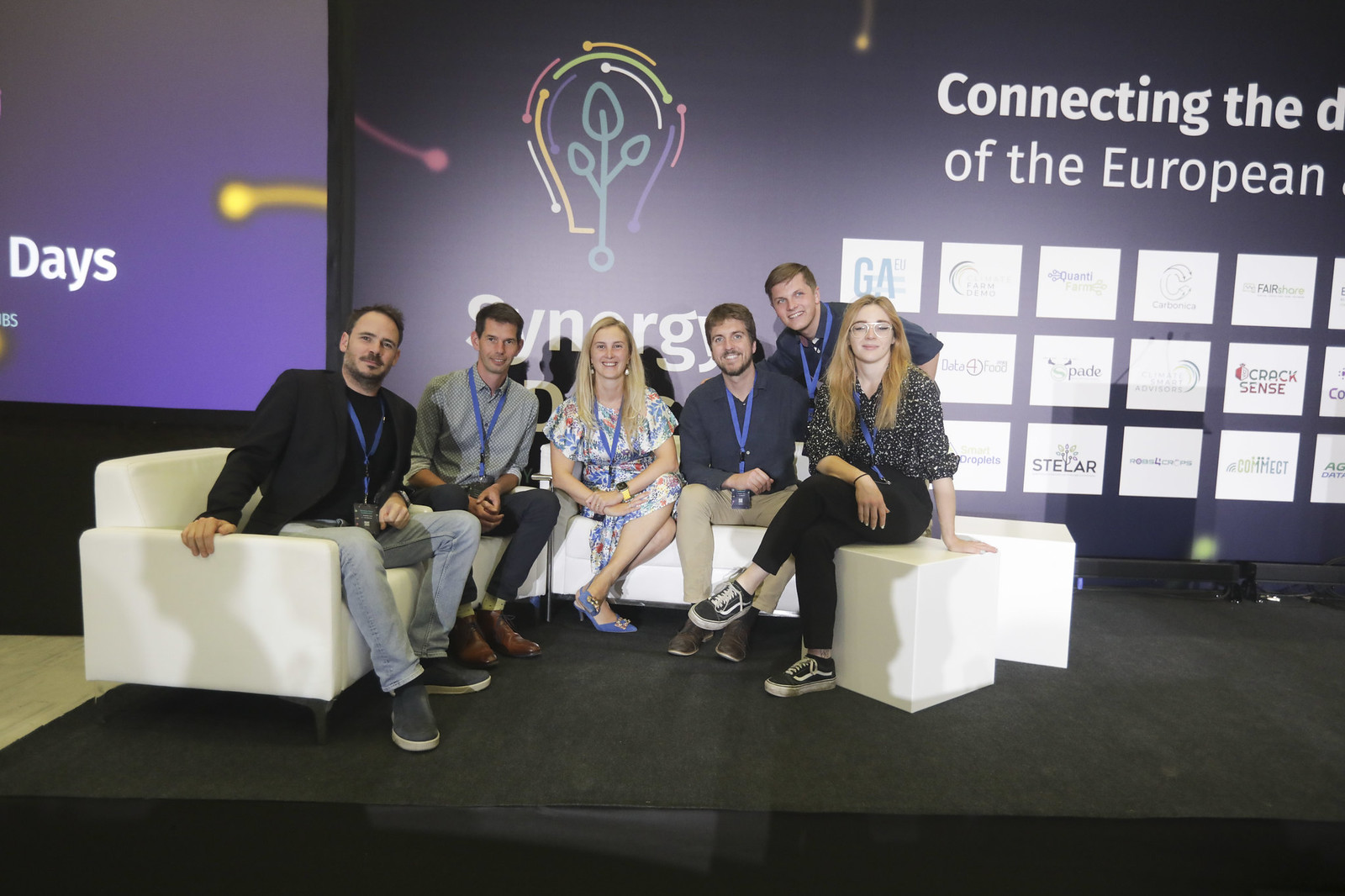This photograph shows a group of six young professionals—two women and four men—posing in a conference room setting, likely during a presentation. They are seated on white couches arranged on a dark gray stage, with one man standing behind the two individuals on the right. All of them are wearing blue lanyards around their necks. The woman in the center is white, blonde, wearing a dress and blue shoes, with her legs crossed. To her left sits a white man in a gray shirt, black slacks, and brown shoes. Next to him is another white man sporting a mustache, clad in a black jacket, blue jeans, and gray sneakers. On the right side of the blonde woman is a man in a black shirt, brown pants, and brown shoes, with another man leaning on his shoulder, also in a dark blue shirt. In the foreground to the right, a white woman with brown or red hair, dressed in black pants and sneakers, sits with her arm resting on a seat, showcasing a bracelet.

Behind the group, the conference room wall is adorned with multiple logos within white squares, and features a colorful light bulb graphic with shades of pink, yellow, green, and purple. A sign in the background reads "Connecting the Dots of the European," suggesting the event's theme, possibly related to school curricula or professional development. The overall ambiance is modern, vibrant, and professional.